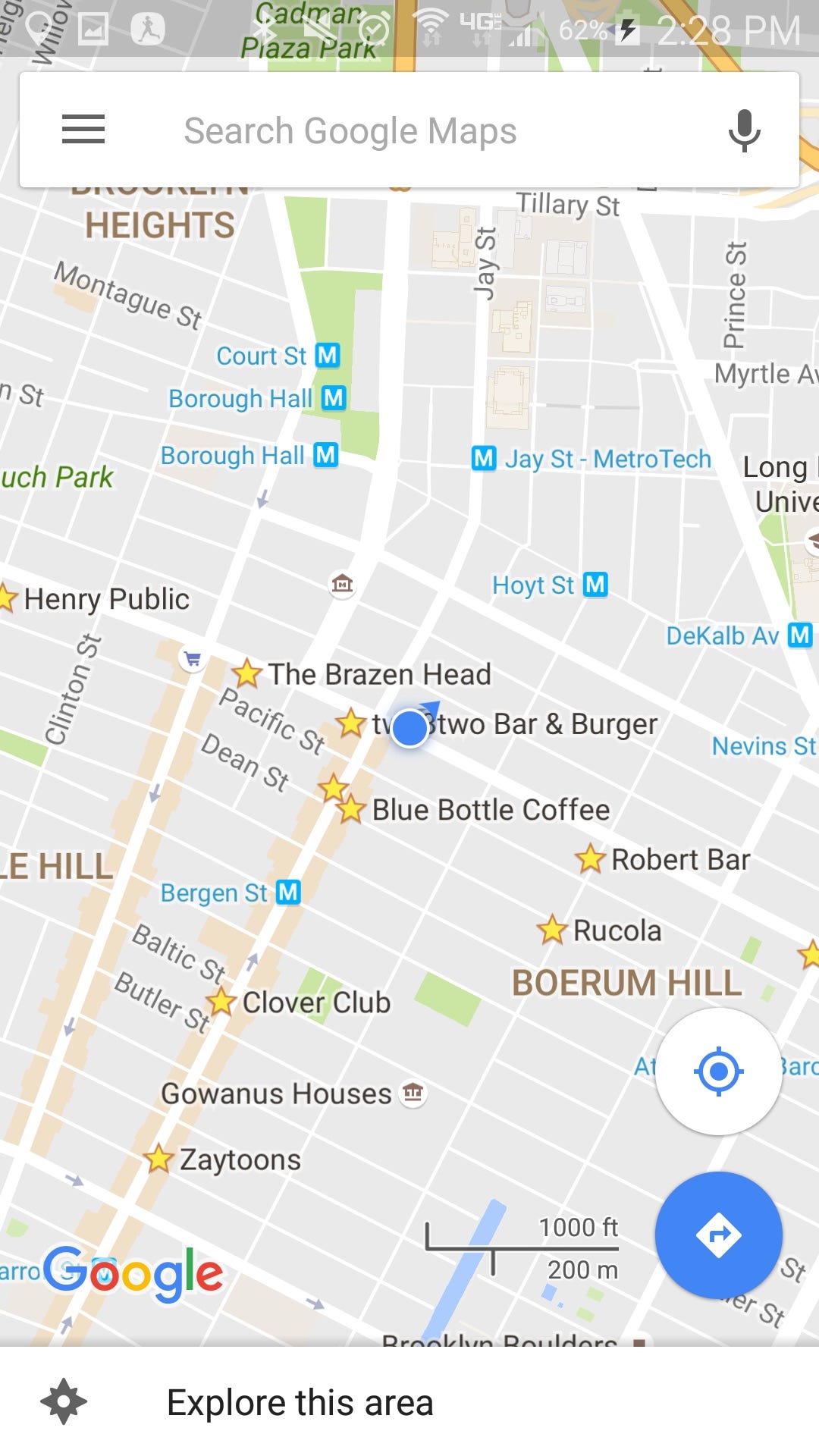This screen capture taken at 2:28 PM shows a smartphone interface with a battery level at 62%, indicated by a black thunder symbol to denote charging. At the top, there's a search bar flanked by a hamburger menu icon on the left and a microphone icon on the right. The main part of the screen displays a map with a central blue circle marked with “The Brazen Head,” depicting a specific location. At the bottom, the Google logo is present. Adjacent to a prominent white circle featuring a blue location symbol is a secondary blue circle with a white diamond inside it, pointing upwards to the right with the text “Explore this area.” Beneath this is a white bar containing a black sun-like icon, adding to the interface’s navigational elements.